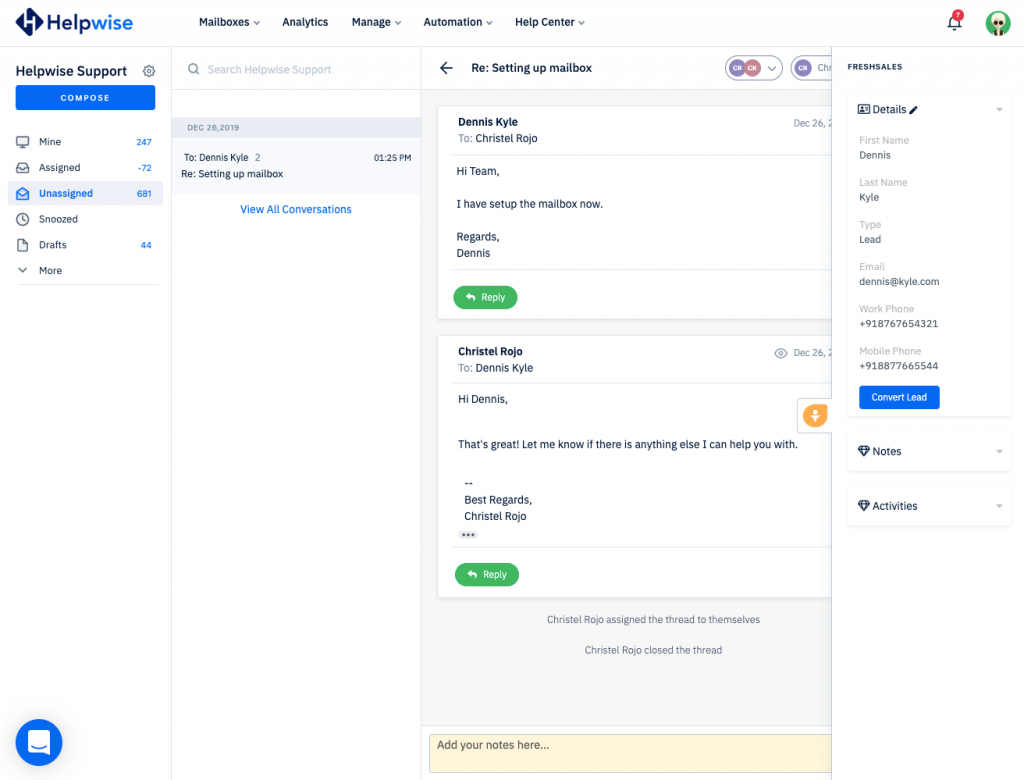This is a detailed screenshot of a help desk interface for "Helpwise Support." At the top-left corner, the label "Helpwise Support" is clearly visible. Occupying a prominent position is a large blue rectangular "Compose" button. Below this button is a list of categories titled "Mine," "Assigned," "Unassigned," "Snoozed," "Drafts," and "More," displayed in black and blue text.

The top navigation menu features options such as "Mailboxes," "Analytics," "Manage," "Automation," and "Help Center." A search bar is available to look through the Helpwise Support system.

The main section showcases an email conversation between Dennis Cow and Crystal Rojo. The first message, from Dennis Cow to Crystal Rojo, reads: "Hi team, I have set up the mailbox now. Regards, Dennis." This is followed by a green "Reply" button. The subsequent reply from Crystal Rojo to Dennis Cow states: "Hi Dennis, that's great! Let me know if there's anything else I can help you with. Best regards, Crystal Rojo," accompanied once again by a green "Reply" button. Additional notations indicate that Crystal Rojo has assigned the thread to herself and then closed it.

At the very bottom, a brown banner invites users to "Add your notes here."

On the right side, a pop-up box titled "Freshsales Details" displays information about Dennis Cow, including his first name, last name, type (Lead), email, work phone, and mobile phone.